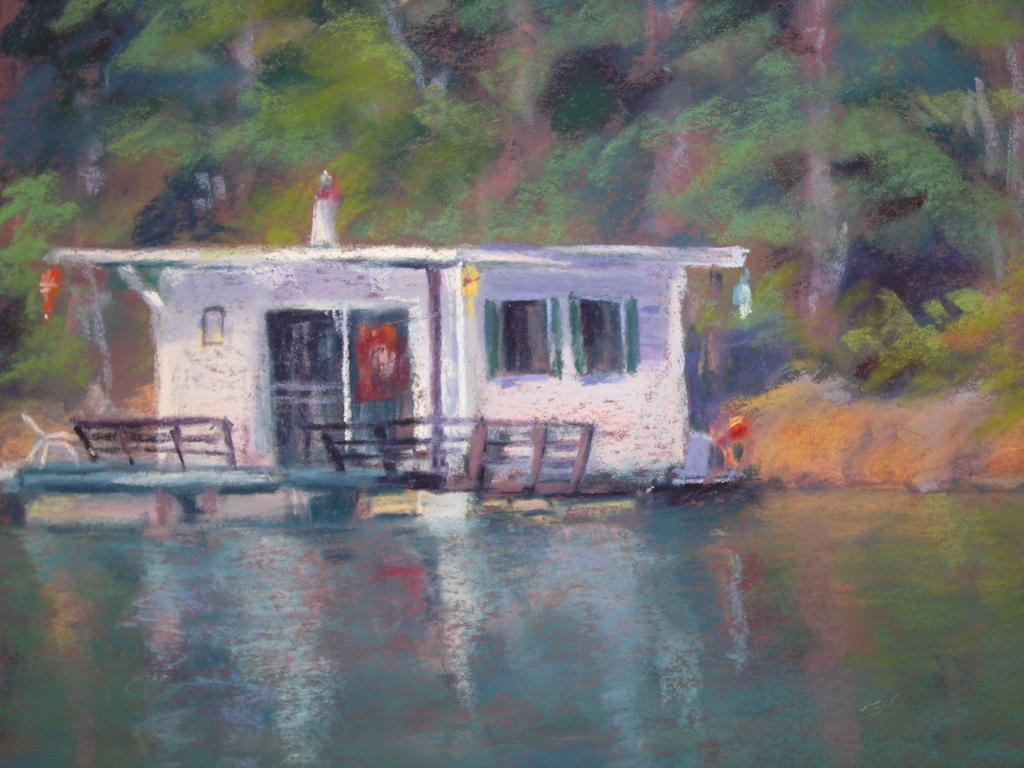The image depicts a muted watercolor painting of a white houseboat floating serenely on a calm, blue-green lake. The houseboat, featuring a porch with brown wooden fencing to prevent falling into the water, nestles closely to the shore, against a verdant backdrop of dense forest. The scene includes subtle and colorful details like a red object and red lights adorning the houseboat. Reflections of the building can be seen on the placid lake surface, further enhancing the tranquil ambiance. The painting shows a realistic touch with possible glimpses of people on the houseboat, indicating life and activity. The range of colors - muted greens, dark greens, light blues, whites, and browns - evoke a peaceful and daytime setting, devoid of harsh shadows, highlighting the brushstrokes' delicate nature across the entire scene.